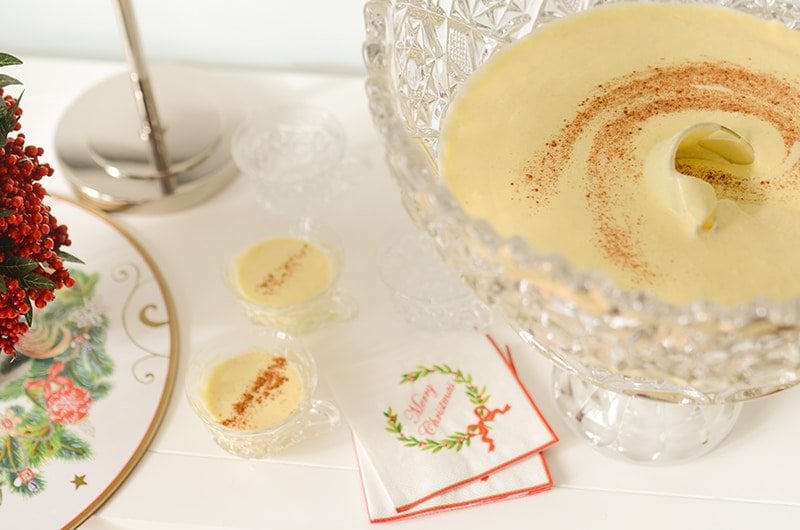This overhead photograph captures a festive, indoor setting centered around a smooth, high-quality, yellow custard-like substance in a clear, crystal-style glass bowl on the right side of the image. The custard, which may indeed be eggnog due to its thicker consistency and holiday-themed context, is topped with a sprinkling of either cinnamon, nutmeg, or brown sugar, forming a delicate swirl on its surface. To the left of the bowl, there are two smaller glass cups, also filled with the same yellow mixture and adorned with similar brown sprinkles. Below these cups, in the middle of the picture, are white napkins featuring a green wreath design with the phrase "Merry Christmas" written inside in red letters. Additional Christmas decorations, such as a plate with a red and green design and a bunch of fake red berries, are visible on the far left, reinforcing the festive theme. Overall, the image exudes a warm and celebratory atmosphere, making it clear that this is a Christmas-themed scene centered around the tradition of eggnog.